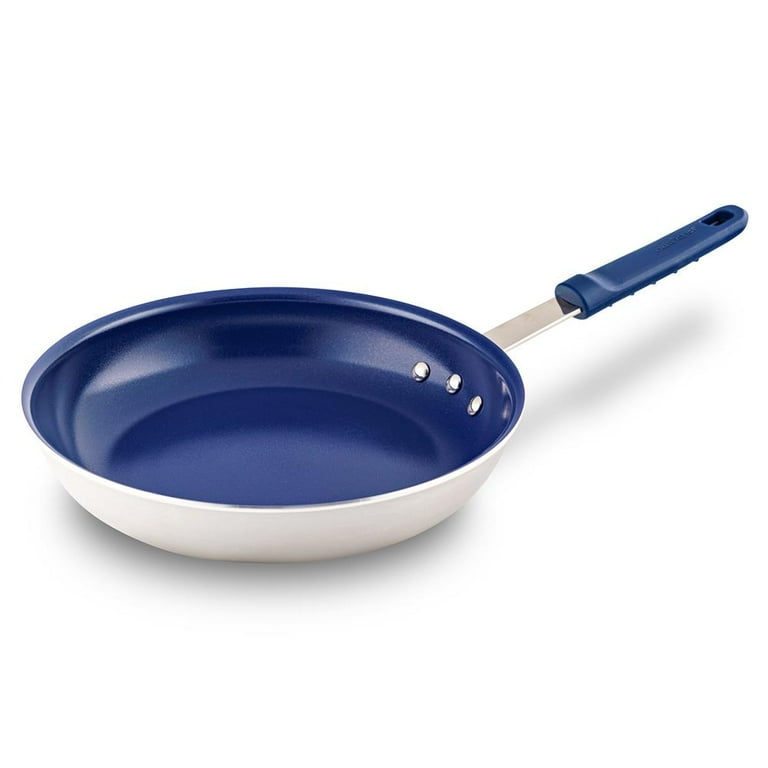The image features a medium-sized frying pan, approximately 10 inches in diameter, set against a plain white background. The interior of the pan is a striking cobalt blue, featuring a protective Teflon non-stick coating that imparts a sparkly finish. The pan's handle is prominently positioned towards the upper right, with the handle itself comprising two distinct parts: a sturdy silver metallic section that connects to the pan via three visible rivets, and a blue plastic grip covering approximately two-thirds of its length, mirroring the interior's color. The exterior of the pan showcases a sleek white or possibly light silver finish, and the overall appearance of the pan is enhanced by its shiny surface, reflecting light at certain angles. Beneath the pan and handle, a subtle gray shadow is visible, adding depth to the otherwise minimalistic background.